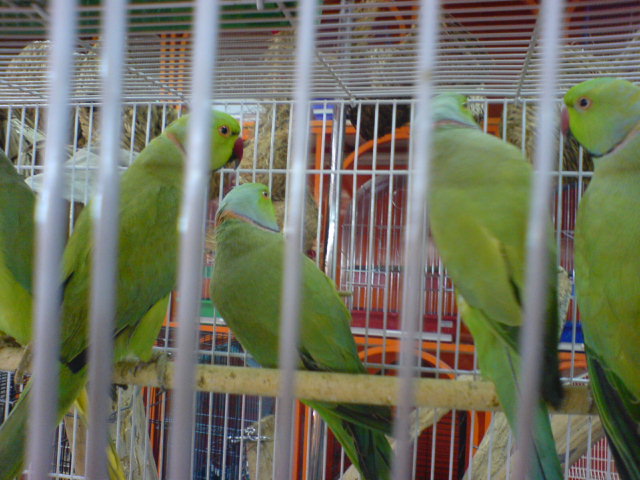This detailed photograph depicts five large, green tropical birds, possibly parakeets or parrots, enclosed within a silver metal birdcage. Their vibrant feathers contrast with darker green wings, round heads adorned with orange eyes, and striking red beaks. Perched mostly on a wooden dowel that stretches horizontally near the bottom of the image, the birds exhibit varied postures: the far-right bird turns its head slightly leftward, showcasing its eye; the second bird faces predominantly away from the camera but glances into the cage; the middle bird’s feet are obscured, as it leans leftward; the fourth bird gazes rightward; and the leftmost bird’s head is out of frame. The cage’s vertical bars, six of which are prominently positioned in the foreground, emphasize the enclosure. Surrounding the scene are other colorful birdcages, hinting at a pet store environment, with hues of blue and orange, wicker baskets, and green trays, creating a bustling ambiance. A glimpse of an orange counter or table adds depth, while food appears to hang within the cage, enhancing the captivity setting.